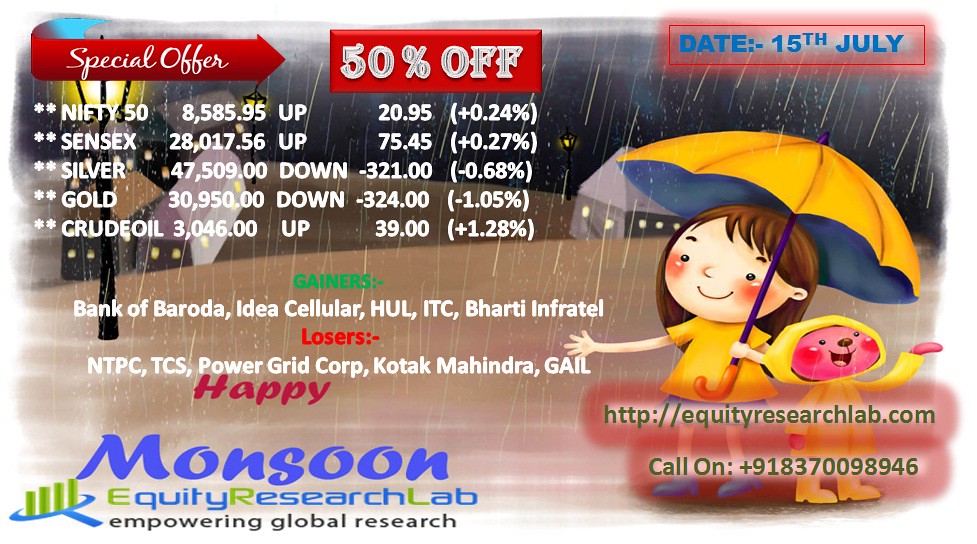The image is a business card-like advertisement for "Monsoon Equity Research Lab," promoting a special offer of 50% off. It is dated 15th July and includes a website, http://equityresearchlab.com, and a contact number, +91 83700 98946. The left side features ticker symbols and prices for various financial instruments, including Nifty 50, Sensex, silver, gold, and crude oil, with their respective performance metrics. Notable gainers and losers in the market are also listed. The right side displays an illustration of a child with brown hair, wearing a yellow shirt, blue skirt, and blue shoes, holding a yellow umbrella, and accompanied by a pink mascot in a yellow raincoat standing on two legs like a human. The text "Empowering Global Research" is prominently featured on the bottom left.